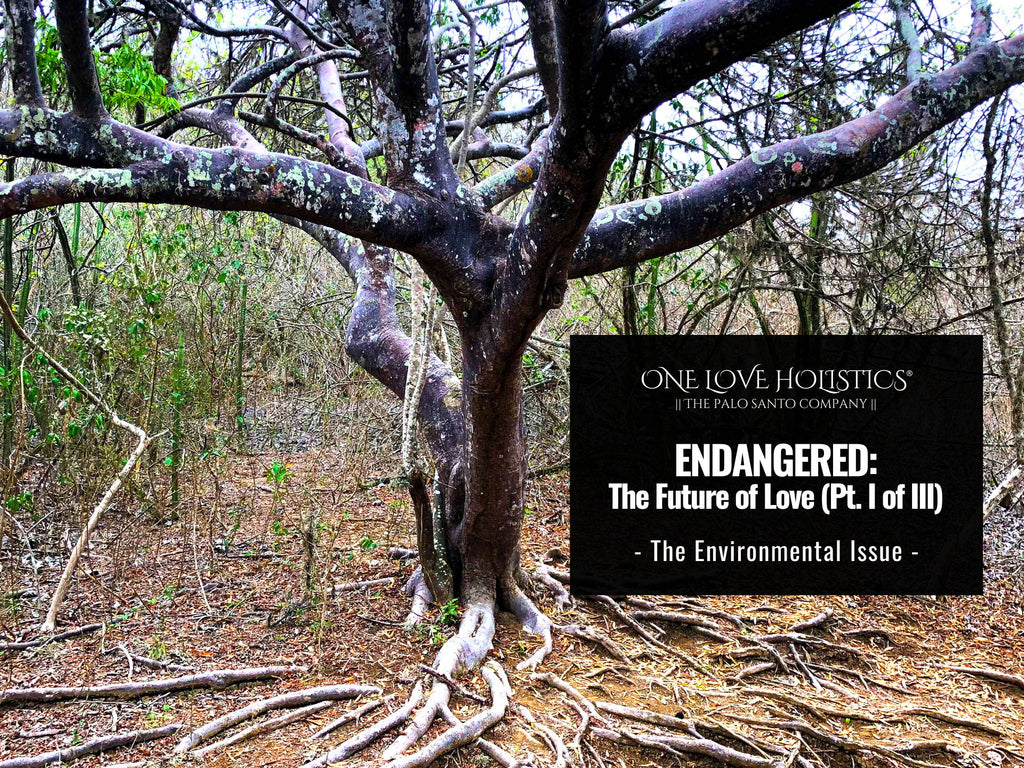In this outdoor photograph taken under an overcast sky, a large, ancient tree commands the center of attention. Its dark, gnarled branches stretch out in various directions, some marked by unusual black, green, and red discolorations that could be moss or other growths. The tree’s root system is notably extensive, with many roots protruding above the ground and fanning out across the dirt and dead leaves that cover the area. In the background, a lush, dense collection of trees and shrubs adds a jungle-like ambiance to the scene. 

A black square appears on the right side of the image, containing white text that reads: "One Love Holistics, The Palo Santo Company, Endangered: The Future of Love (Part 1 of 3), The Environmental Issue." This element suggests the image serves as an advertisement or promotional material, likely highlighting the environmental plight of both the tree and the broader ecosystem it represents. Despite the visible distress on the tree, indicating potential environmental struggles, the overall setting is rich with vegetation, reinforcing the urgent message conveyed by the text.